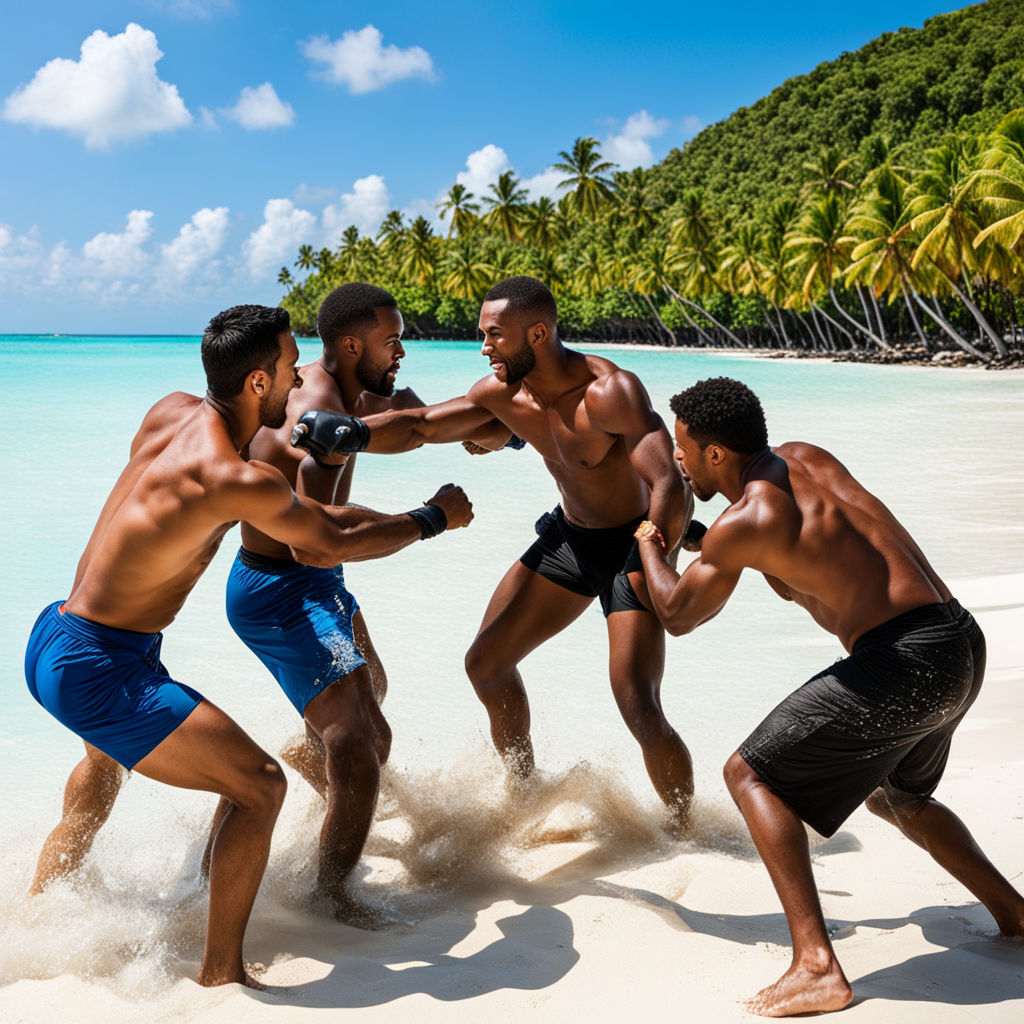In a serene yet dynamic beach scene, a highly detailed and photorealistic painting portrays four muscular African-American young men engaged in a playful fight or exercise, reminiscent of wrestling or boxing. Two men on the left don blue swim trunks while the two on the right wear black trunks. The man in the center, who wears black trunks, has a boxing glove on his right hand, poised in an upward fighting stance. Directly facing him to the right, another man in black trunks is bent over defensively. The setting is idyllic, with their bare feet buried in the soft sand that meets the edge of a luminescent aqua-blue ocean. The sky above is a clear blue, adorned with wisps of white clouds, and the left side of the background showcases a lush forest filled with green trees, while the right side reveals towering palm trees, suggesting an island paradise. The digital quality of the image lends a slightly surreal, almost AI-generated aesthetic to the men, enhancing the photorealistic effect of this vibrant and energetic beach tableau.